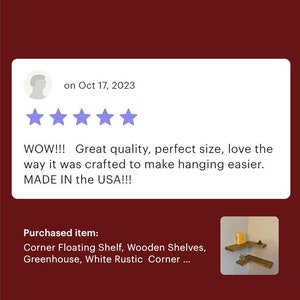This image showcases a cropped screenshot of a customer's review on a handcrafted item. The background is a rich burgundy color. At the top left of the screenshot is a blank profile picture circle. To the right of the profile picture, the date "October 17th, 2023" is displayed in small purple letters. Below the date are five large purple stars signifying a five-star rating.

The review reads: "Wow, great quality, perfect size, love the way it was crafted to make hanging easier. MADE IN THE USA!!!"

Beneath the comment box, on the left side, there's a description of the item purchased: "Corner floating shelf, wooden shelves, greenhouse, white rustic corner..." To the right of this description is a small square thumbnail showcasing the shelves floating on the walls.

Overall, the image highlights positive feedback on the quality and design of the corner floating shelf, emphasizing its ease of use and thoughtful craftsmanship.